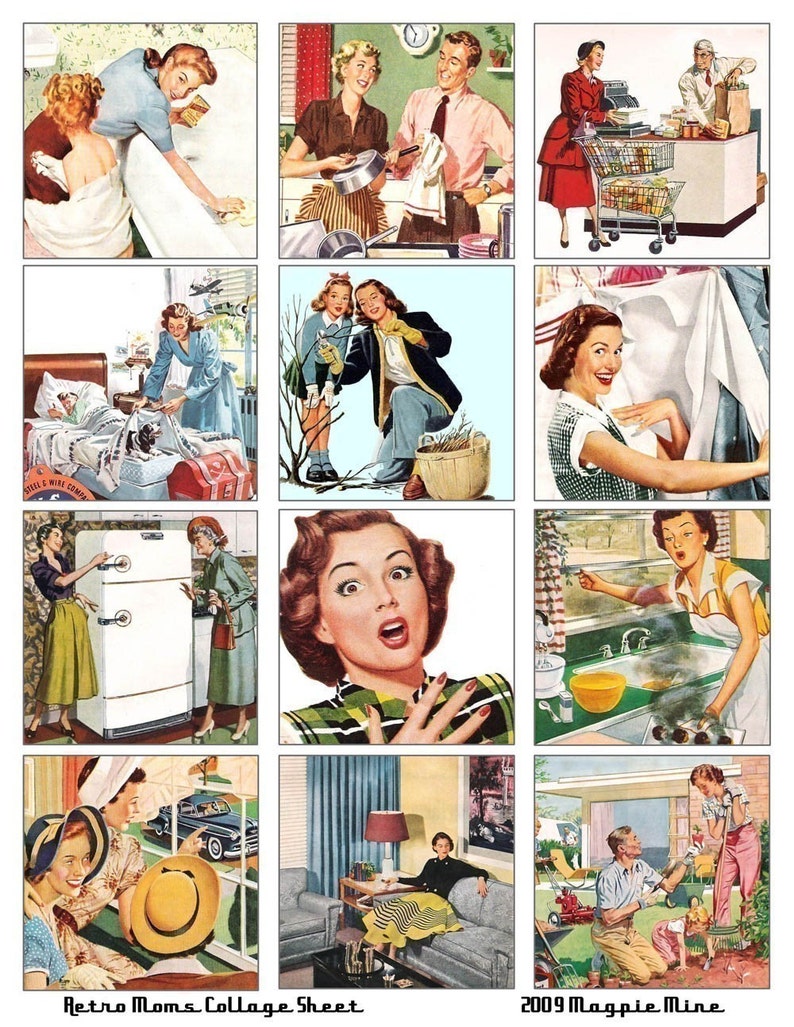This retro collage, titled "Retro Mom's Collage Sheet," consists of twelve hand-drawn, vibrantly colored illustrations laid out in a three-column by four-row grid, reminiscent of 1950s magazine art. Each image captures different domestic scenes featuring a housewife performing typical chores and activities of the era. 

In the top left, a mother scrubs a bathtub while her daughter, wrapped in a towel, steps out from taking a bath. Adjacent to this, the next picture shows a couple in the kitchen; the woman dries a pan while the man assists with a drying towel. In the third image, a woman is seen at the grocery store, conversing with the cashier as he bags her groceries.

Additional scenes include a mother tucking a dog into bed with her sleeping child, teaching her daughter gardening in the backyard, hanging laundry on a clothesline with a joyful expression, and chatting with an elderly lady dressed in green in front of a refrigerator. Another detailed drawing portrays a woman gasping as she's burnt something on the stove, wisps of smoke rising while she opens a window.

The bottom row features three women, one with her back turned wearing a yellow hat as they look out at a 1960s car. Another image captures the woman taking a break on a gray couch, surrounded by blue curtains and a piece of artwork hanging on the wall. The final panel shows the diligent housewife engaged in yard work alongside a man holding a red pepper and a child digging in the dirt.

Combining elements of comic strip aesthetics and nostalgic pin-up art, this 2009 creation by Magpie Mine encapsulates the essence of a 1950s housewife's daily life in vibrant detail and vintage fashion.